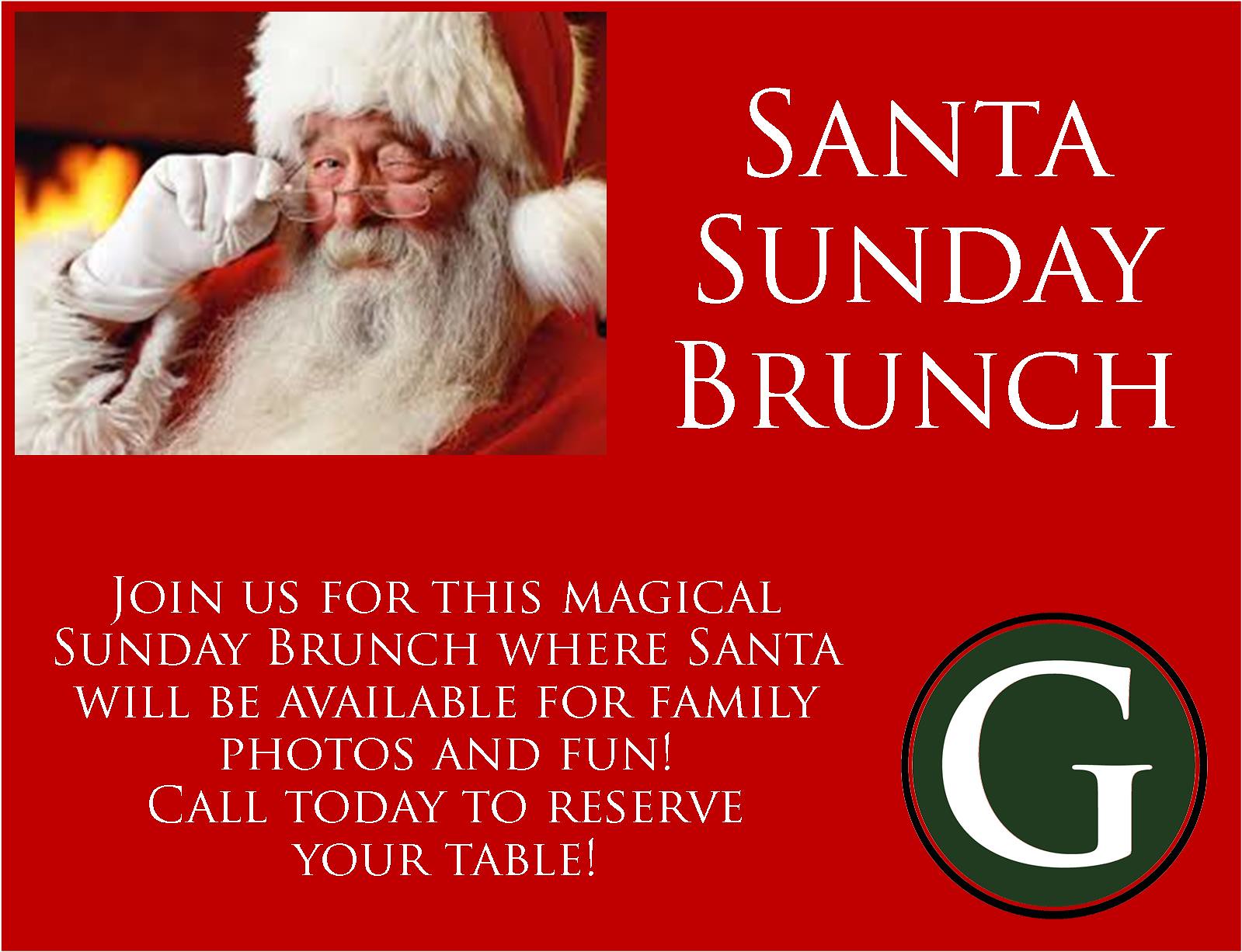The image appears to be a digitally crafted invitation for a festive event named "Santa Sunday Brunch." It features a rich red background with all text in white capital letters. On the top left corner, there's an image of Santa Claus, depicted with a full grey beard, red hat with white fur trim, white gloves, and glasses he is playfully pulling down while winking. To the right of Santa's image, the text reads "SANTA SUNDAY BRUNCH." Beneath this, it states, "Join us for this magical Sunday Brunch where Santa will be available for family photos and fun. Call today to reserve your table." On the bottom right corner, there is a green circular icon featuring a capital 'G' in white. Overall, the image invites families to a special brunch event with Santa, promising photo opportunities and fun activities.